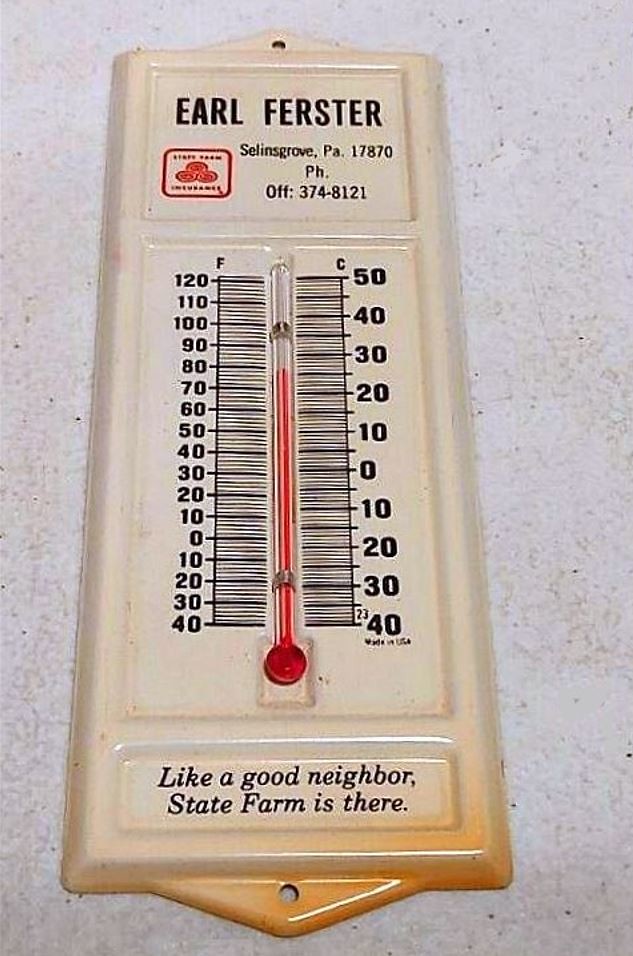This is a detailed vertical color photograph of a vintage State Farm Insurance representative thermometer. The thermometer is made of flat metal with slightly raised edges and features nail holes at the top and bottom for mounting. At the top, it prominently displays the name "Earl Furster, Selling Grove, Pennsylvania, 17870" along with the office phone number "374-8121." This off-white thermometer, which transitions to a more orange hue at the bottom, appears to be aged, possibly with some fading of its original colors. The black typeface stands out against the background, ensuring readability.

In the middle section, a red mercury thermometer encased in glass is flanked by temperature scales. On the left side, the Fahrenheit scale ranges from -40 to 120 degrees, while on the right side, the Celsius scale ranges from -40 to 50 degrees. Toward the bottom of the thermometer, the classic slogan "Like a good neighbor, State Farm is there" is printed, emphasizing its promotional nature as a giveaway item.